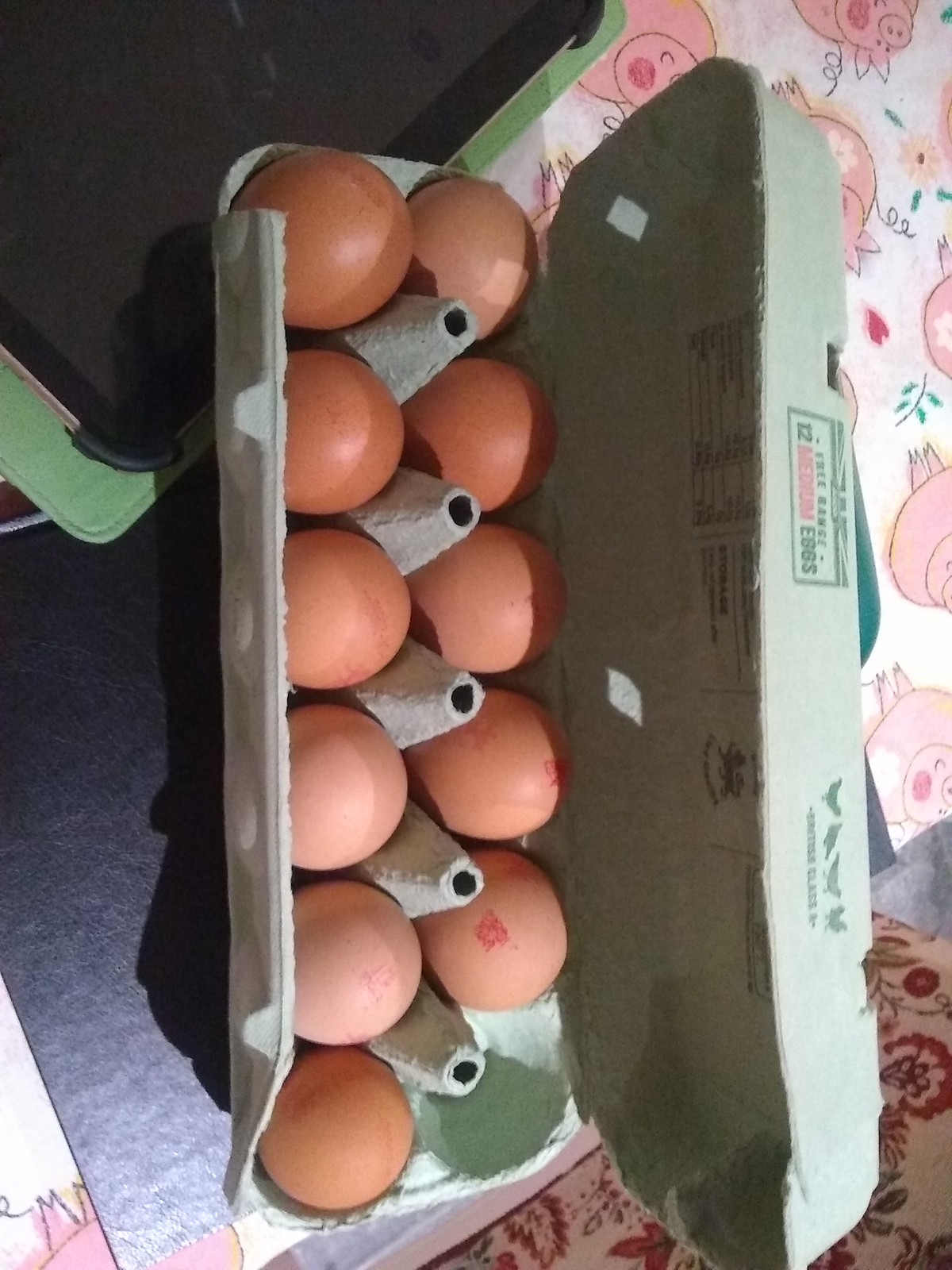The image shows an open, lengthwise egg carton made of bluish-gray cardboard containing 11 brown eggs, some of which are stamped with a red mark that appears to be in Chinese. The carton, bearing the label "12 medium eggs" along with an illustration of four chickens and a rooster, and nutritional information is printed on the inside flap. The eggs are nestled in pointed inserts with holes on top. The carton lies on a black surface, possibly a cutting board or placemat, which rests on a table covered by a tablecloth adorned with cartoon pigs, branches, and hearts. Adjacent to this setup, part of the table is covered with a paisley print cloth in dark red, maroon, and green hues. Additionally, a green electronic device, likely an iPad or its case, is visible at the top of the image.